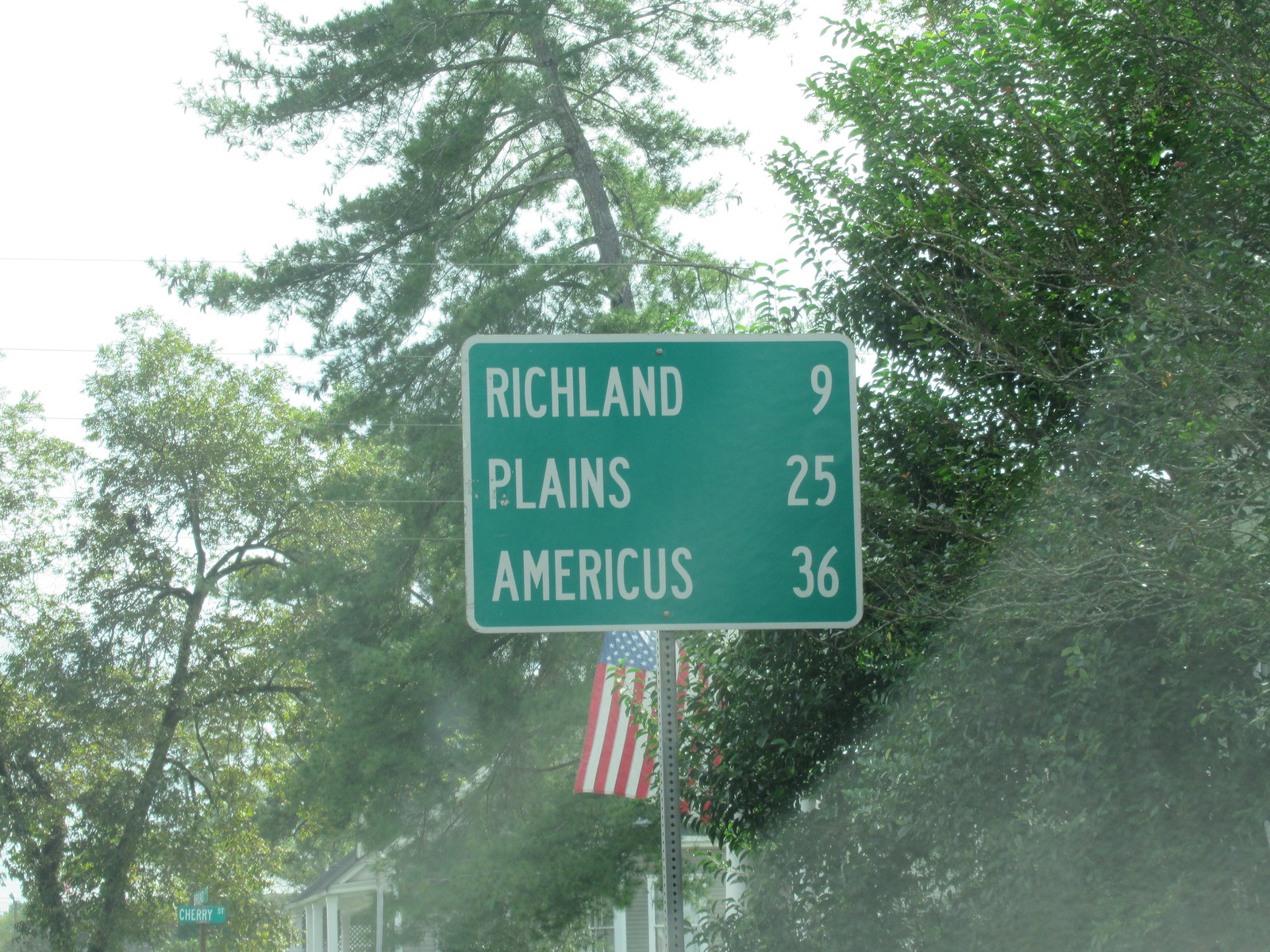The image features a prominent green street sign with white lettering, situated next to a cluster of trees. The sign displays directional information: "Richland - 9 miles," "Miles Plains - 25 miles," and "America - 36 miles," though the name of the road it is on is obscured. To the right of the sign, there is a tall, lush green tree, with a slightly taller tree leaning to the left behind it. Below these trees, an American flag is partially visible, its view hindered by the sign and branches.

In the background, there are a few houses with white porches and what appear to be gray roofs, though the roofs are largely obscured by the surrounding trees. The scene is clearly somewhere in America, adding context to the flag. Overall, the street sign, with its green background and white text, serves as the focal point of the image, drawing the viewer's attention amidst the natural and architectural elements around it.